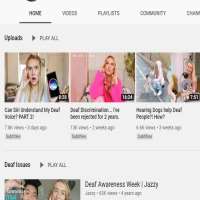This screenshot captures a portion of a website, specifically a segment of the menu and video thumbnails. The header is truncated, leaving the website unidentified, though the interface suggests it could potentially be TikTok. The partial menu strip includes options such as Home, Videos, Playlist, and Community. The scene is dominated by a white background, with all text rendered in black. 

At the top of the image, a section labeled "Uploads" is prominently displayed. Below this, there are three video thumbnails arranged horizontally, though the text accompanying these thumbnails is small and blurry, making it difficult to discern details. Toward the bottom of the screenshot, the category "Deaf Issues" is highlighted, accompanied by an option to 'Play All'. One of the visible video titles is "Deaf Awareness Week," which appears at the top of this collection of thumbnails. 

This depiction offers a glimpse into a website page that is focused on video content related to Deaf awareness and issues.